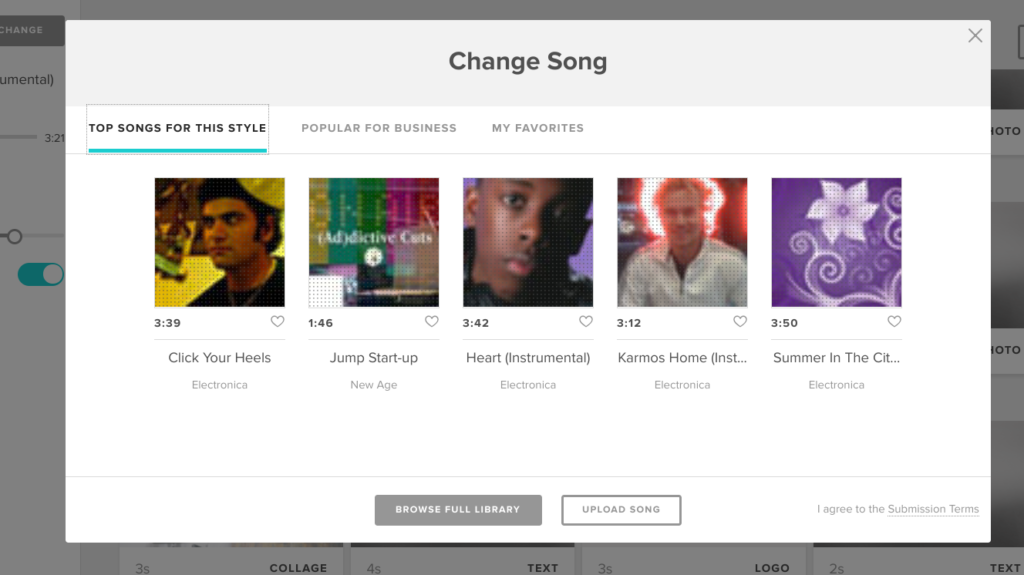The image is a screenshot of a playlist featuring various songs. At the top of the screenshot, the text "Change Song" is prominently displayed, followed by the phrase "Top Songs for This Style," both written in black with a turquoise underline. Below this section, "Popular for Business" and "My Favorites" are indicated in gray text.

The playlist includes several songs with distinctive attributes:

1. "Click Your Heels" - An electronica track with a duration of 3:39. This song is marked with a heart symbol indicating it is favorited. The cover image features a man set against a yellow background.

2. "Jumpstart" - A new age song that has also been marked as a favorite, with 146 listed beside it. The cover image displays a vibrant mix of colors, including blues and pinks.

3. "Heart Instrumental" - An electronica track featuring an image of a Black man looking directly at the viewer. 

4. "Carmo's Home" - Another electronica song with a cover image showing a white man wearing a white jacket, surrounded by an electric aura around his head.

5. An unnamed electronica track with a purple aesthetic, highlighted by a purple flower in the cover image.

Overall, the playlist is a curated selection of electronica and new age tracks, each with visually distinctive cover art and unique attributes.